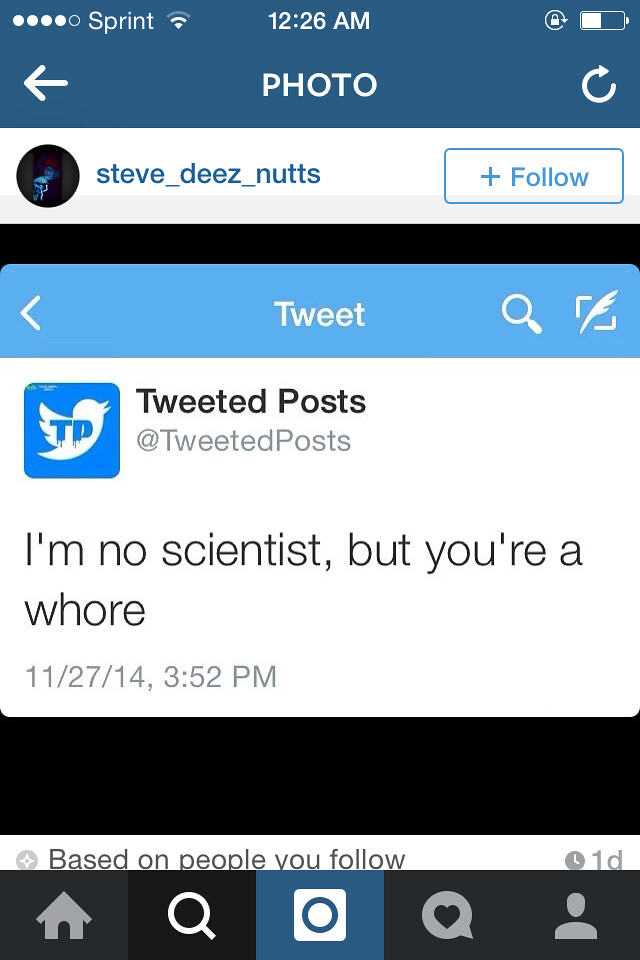A detailed screenshot of an iOS device, specifically displaying the Instagram app open on a Sprint mobile network at 12:26 AM. The battery level is about halfway. At the top, the dark blue bar includes a back arrow, the title "Photo", and a refresh button on the right. Below, the account being viewed is Steve_D's_Nutts, with a hollow "Follow" button next to the username. The main content of the screenshot is a reposted tweet, which is displayed on a white background with black text. The tweet, originally posted on November 28, 2014, at 3:52 PM by Steve_D's_Nutts, reads, “I'm no scientist, but you're a whore.” Beneath this, there is a black bar with text indicating "Based on people you follow." At the very bottom, the standard Instagram navigation bar is visible, featuring buttons for home, search, camera, notifications (a speech bubble with a heart in it), and the profile page.